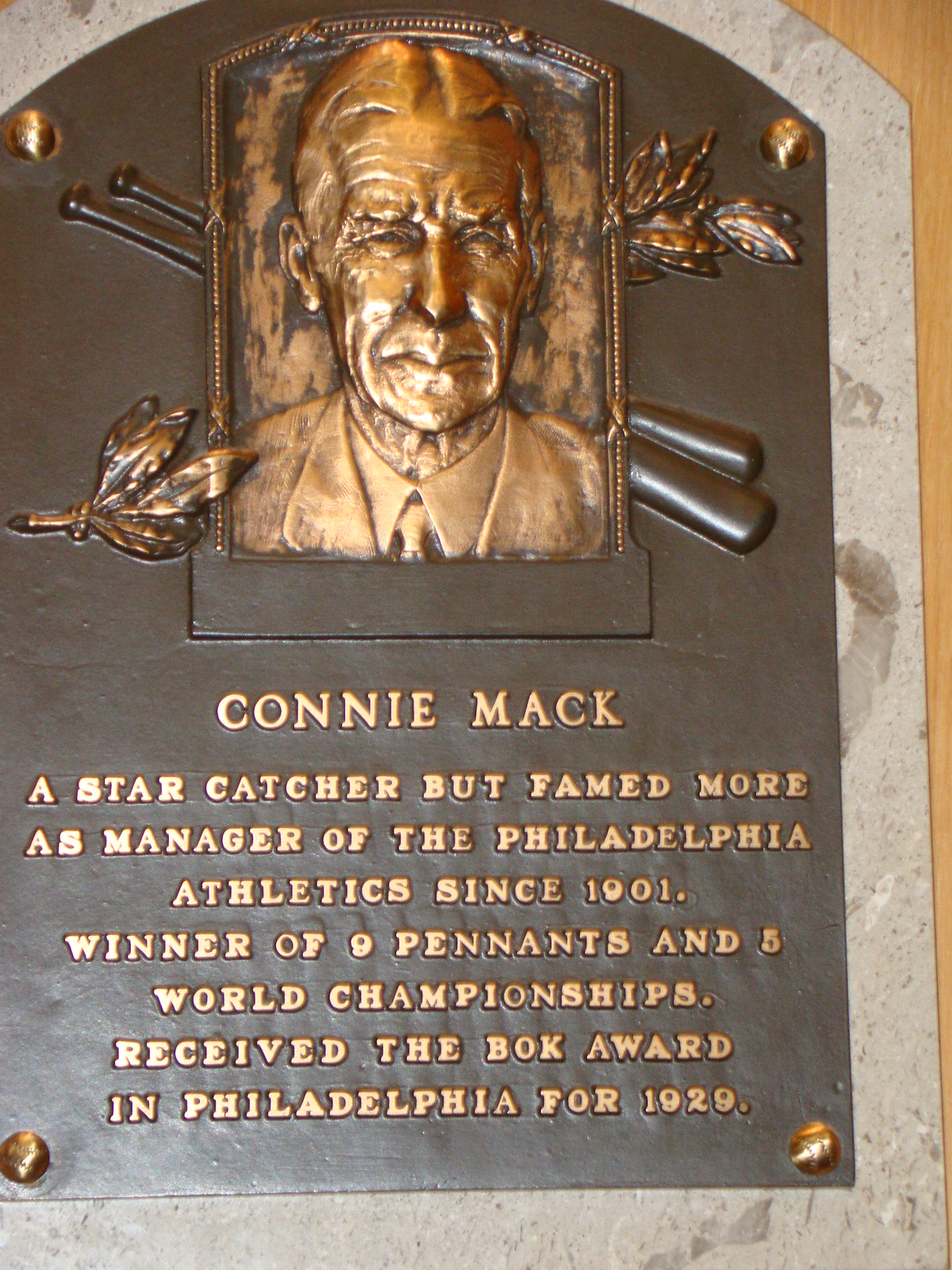The image depicts a detailed memorial plaque dedicated to Connie Mack, noted baseball manager and former catcher. The plaque is mounted on a marble wall and features a bronze relief of Connie Mack's face, framed by two baseball bats and a surrounding motif of leaves. The plaque itself has a brown center bordered by gray, and brass with lighter, rubbed highlights. The text on the plaque reads: "Connie Mack, a star catcher but famed more as manager of the Philadelphia Athletics since 1901. Winner of nine pennants and five world championships, received the BOK Award in Philadelphia for 1929."